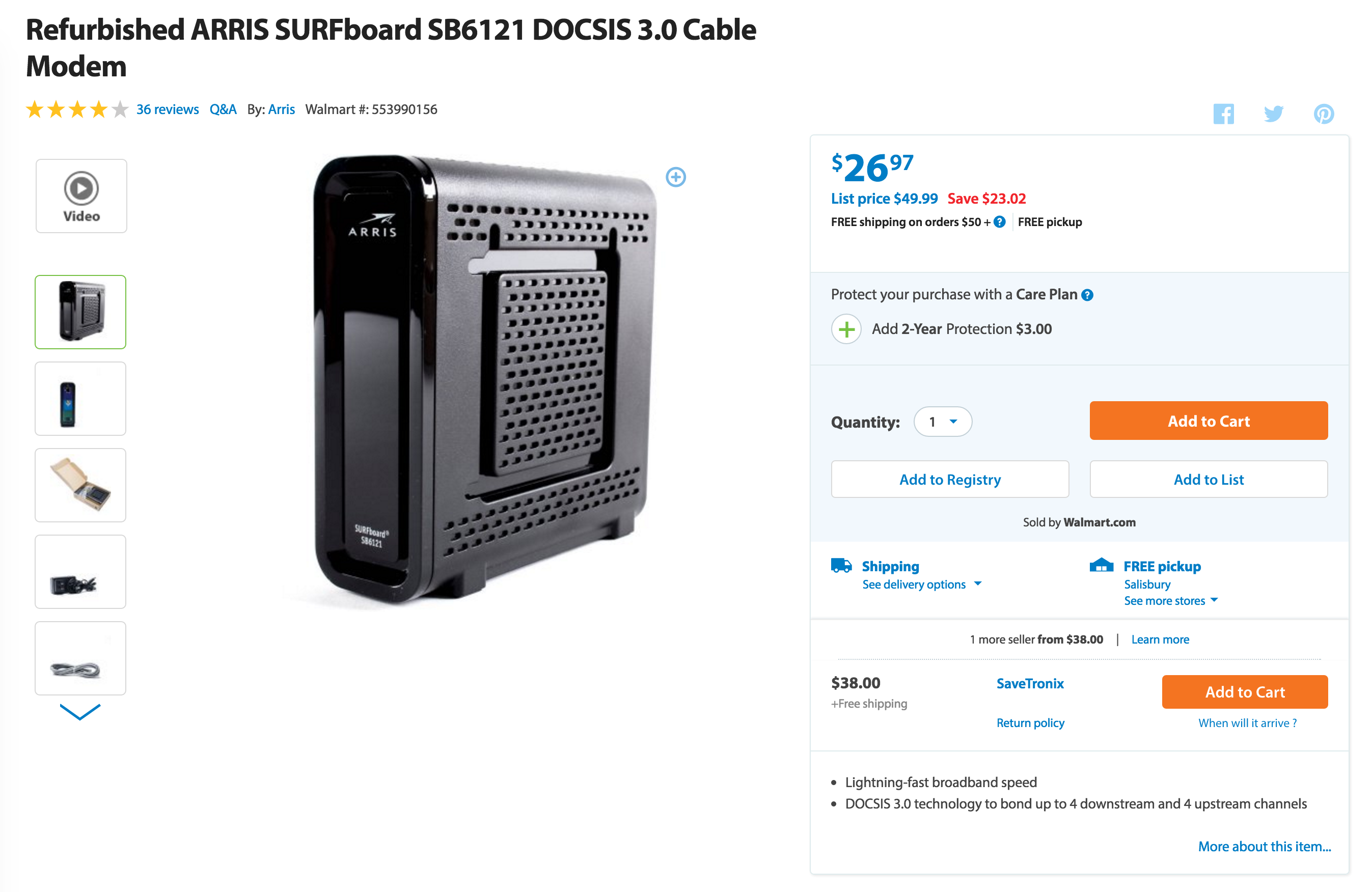**Screenshot of a Website Product Page for Refurbished ARRIS SURFboard SB6121 DOCSIS 3.0 Cable Modem**

The image captures a product page on a website with a clean white background. At the top-left corner, the product title is displayed in bold black text: "Refurbished ARRIS SURFboard SB6121 DOCSIS 3.0 Cable Modem," with "Modem" moved to the next line for left justification. 

Directly beneath the title are product icons and ratings. The item has a four out of five-star rating, with four gold stars and one gray star on the far right. Next to the star rating, blue text indicates "36 reviews Q&A," with "Buy: ARRIS" in blue text and followed by "Walmart number 553-99-0156" in black text.

Below this section are preview images aligned to the left and bounded by thin gray outlines. Each preview image has a white background. The topmost preview features a gray circle with a white triangle pointing to the right, indicative of a video. Below this icon is the word "Video" in gray text.

The next preview image, highlighted with a green outline to show it's selected, displays a black modem. This same black modem is prominently featured in an enlarged form to the right, covering the same height as the preview images.

Further down, the third preview image depicts a black rectangle with a blue section. The fourth image shows a light beige open box containing the black modem. The fifth preview showcases a wrapped charging cable, while the last image displays a gray ethernet cable.

To the right of the enlarged modem image, the product information, including the price, is presented.